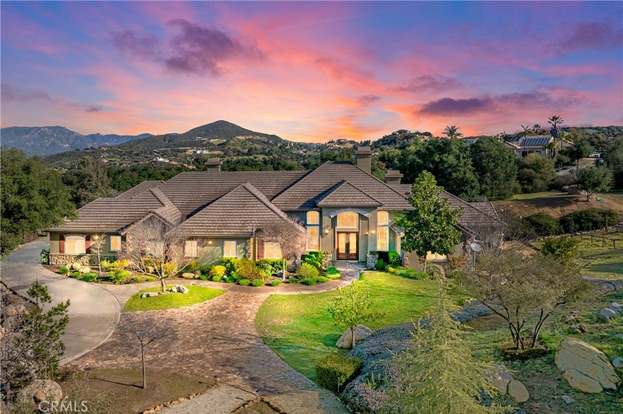This illustration depicts a fairly large, prominent home, possibly a mansion, characterized by its intricate architectural design with multiple wings and varying roof lines. The roofs are gray, and there are several chimneys suggesting a two-level structure, emphasizing its prominence. The front view reveals a sprawling, elaborate garden filled with bushes, small trees, and meticulously arranged rocks. A large twisty path leads to the entrance, while a driveway curves around the left side of the house. The lawn on the right is well-manicured with additional trees and rocks, and the garden extends prominently into the foreground. The background features a backdrop of hills or mountains, and the sky bursts with shades of orange, purple, and blue, adding a dramatic touch to the scene. The image, devoid of any people, appears serene and well-maintained, and in the bottom left corner, the text "CRMLS" is visible. The numerous windows of the house allow light to pour through, enhancing its inviting and grand appearance.